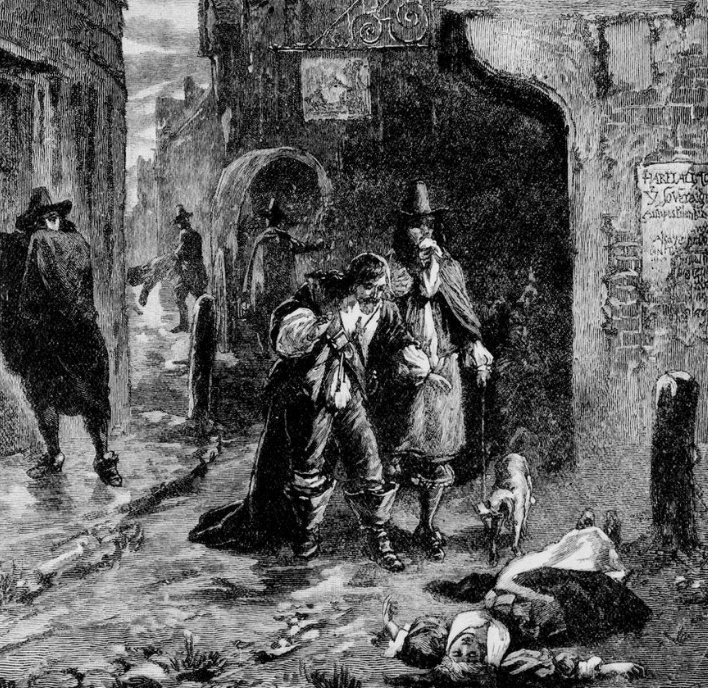The black and white illustration, possibly an etching or pen and ink drawing, evokes the atmosphere of a bygone era, likely the 1800s or early 1900s. The scene is set in a dimly lit alleyway flanked by brick buildings adorned with tattered posters, adding to the dramatic ambiance. At the center of the image, a woman lies reclined, possibly dead or unconscious, on the cobblestone street. Two men, dressed in elaborate, old-fashioned attire with boots and long robes, stand over her. One man, who has a goatee and longish hair, clutches a sword across his chest and holds a handkerchief over his nose and mouth. The other man appears to be blind, wearing dark glasses and a wide-brimmed hat, with a cape draped over him. Near the woman's legs, a small dog stands, seemingly alert. To the left, another man in a dark hat and glasses covers his face with his arm or cape, adding to the scene's tension. In the background, the image fades into darkness, but a covered wagon and additional onlookers can be vaguely discerned, contributing to a tunnel-like effect that heightens the sense of depth and mystery.